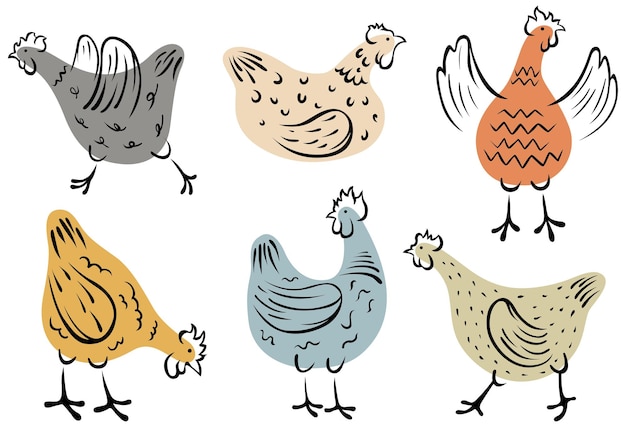The image depicts a set of six graphically designed chickens set against a white background, organized in two rows of three. The chickens are cartoonishly illustrated with clear combs, beaks, and wings. The top row features a gray chicken at the left, facing left with its wings raised; a peach-colored chicken lying down facing right; and an orange-brown chicken with raised wings in the far right position, also facing right. On the bottom row, the leftmost chicken is yellow-brown, pecking at the ground; the middle chicken is light blue and standing while looking backwards over its shoulder to the left; and the rightmost chicken is a darker lavender shade, walking to the left. Each chicken features unique patterns such as diagonal lines, zigzags, and spots resembling leopard prints.